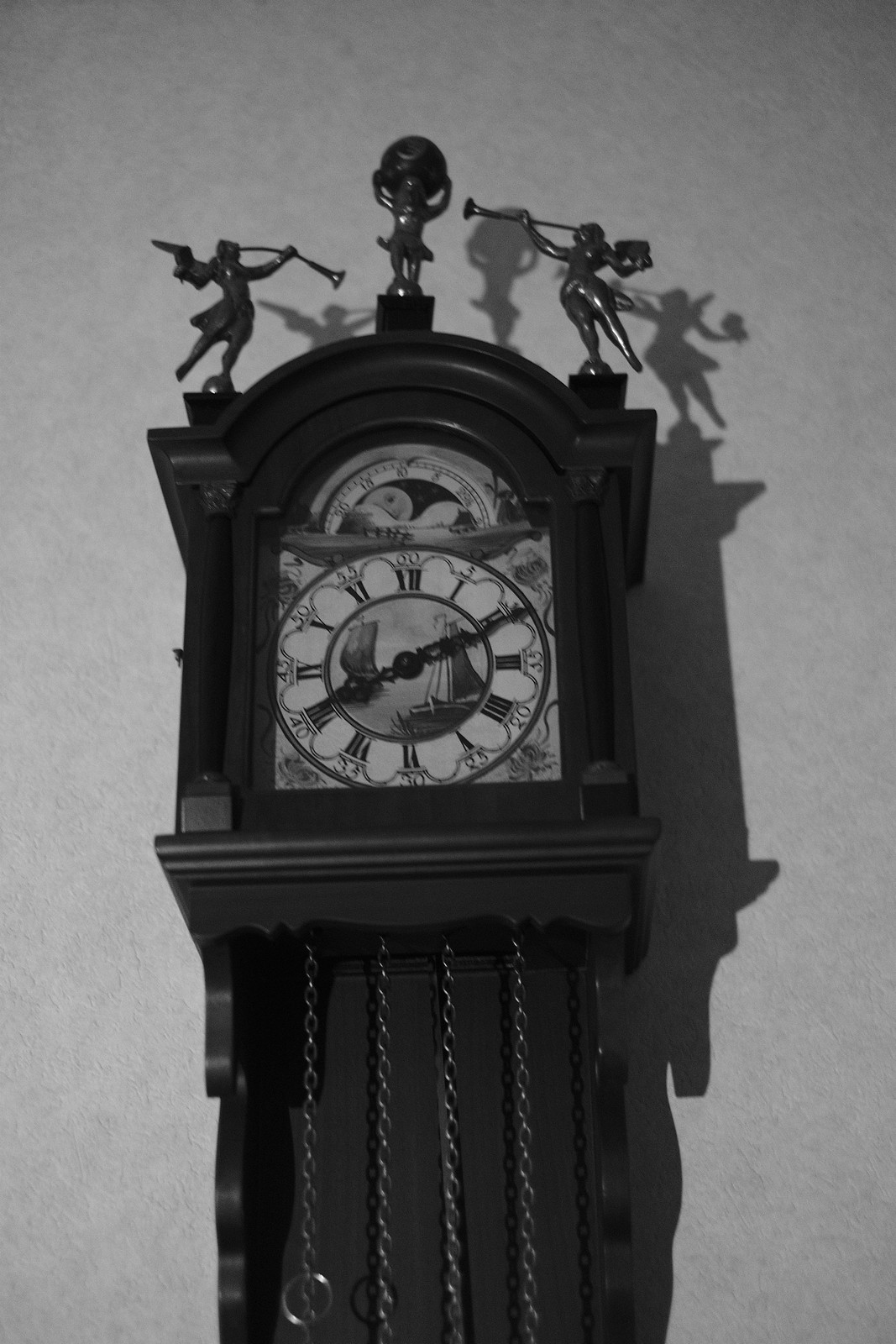This monochromatic photograph captures a beautifully intricate vintage grandfather clock, likely of significant value. The image is taken from a low angle, creating a sense of towering majesty as it forces the viewer to look up at the clock. Perched atop the clock are three statues: the ones on the left and right are depicted blowing trumpets, while the central statue is shown lifting a globe or the Earth on its shoulders, adding an air of classical grandeur.

The clock face is adorned with Roman numerals, contributing to its antique charm. At the center of the clock face, there are two ship illustrations, suggesting themes of exploration and adventure. Above the ships, an illustration of the moon with a human-like face adds a whimsical and celestial touch. The overall composition, combined with the black-and-white scheme, imbues the photograph with a timeless, almost mystical quality.